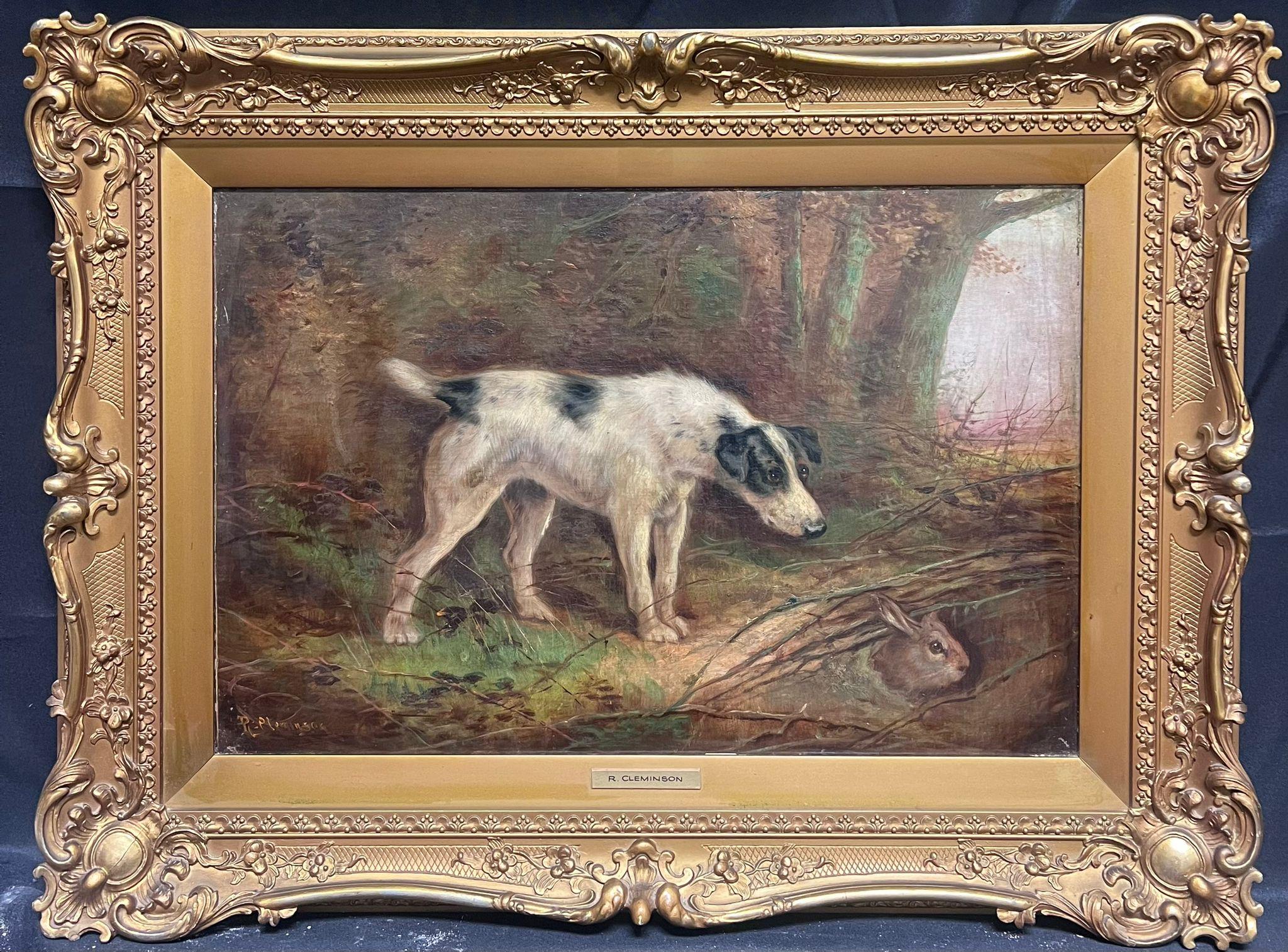The painting, titled "Terrier's Ratting" by R. Cleminson, is displayed in an extraordinarily ornate, matte gold frame that features intricate scroll work, 3D bevels, and floral moldings, adding to its luxurious appearance. The scene within this opulent frame captures a predominantly white dog with black spots, including around its eyes, back, and near the tail, standing in pointer fashion at the base of a tree within a thicket. The dog, which stands on a blend of brown and green grass amidst a marsh or bog-like setting, intently focuses on a small brown rabbit peeking out of a hole nestled in the roots of the tree. The background showcases a dense cluster of leafless trees, painted with orange hues that suggest an autumnal setting. The detailed and lifelike depiction of the dog and its natural surroundings creates a captivating and dynamic scene, aptly highlighted by the lush and vividly textured frame.